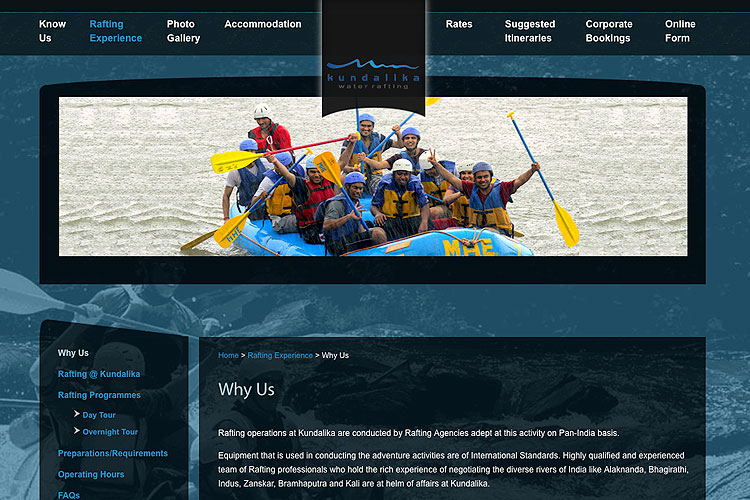Here is the cleaned-up and detailed caption:

---

This is a screen capture in portrait mode showcasing the website for Kundalka Water Rafting. At the top of the screen, a navigation menu features several options, including "Know Us," "Rafting Experience" (highlighted in blue to indicate the current page), "Photo Gallery," "Accommodation," "Rates," "Suggested Itineraries," "Corporate Bookings," and "Online Forum." 

Below the menu, there is a wide photograph displaying a group of enthusiastic rafters in an inflatable raft, all smiling at the camera with their paddles raised high. The background features another image, partly visible, filled with more rafting activity, emphasizing the adventurous vibe of the website.

On the left side of the screen, there is a section titled "Why Us" in a black background with blue fonts. It includes subcategories such as "Rafting Programs," "City or Day Tour," "Overnight Tour," "Preparation Requirements," "Operating Hours," and "FAQs."

To the right, there is a breadcrumb navigation trail starting with a cookie icon, followed by "Home," "Rafting Experience," and "Why Us." Below this, a paragraph elaborates on the reasons to choose Kundalka for your rafting experience.

---